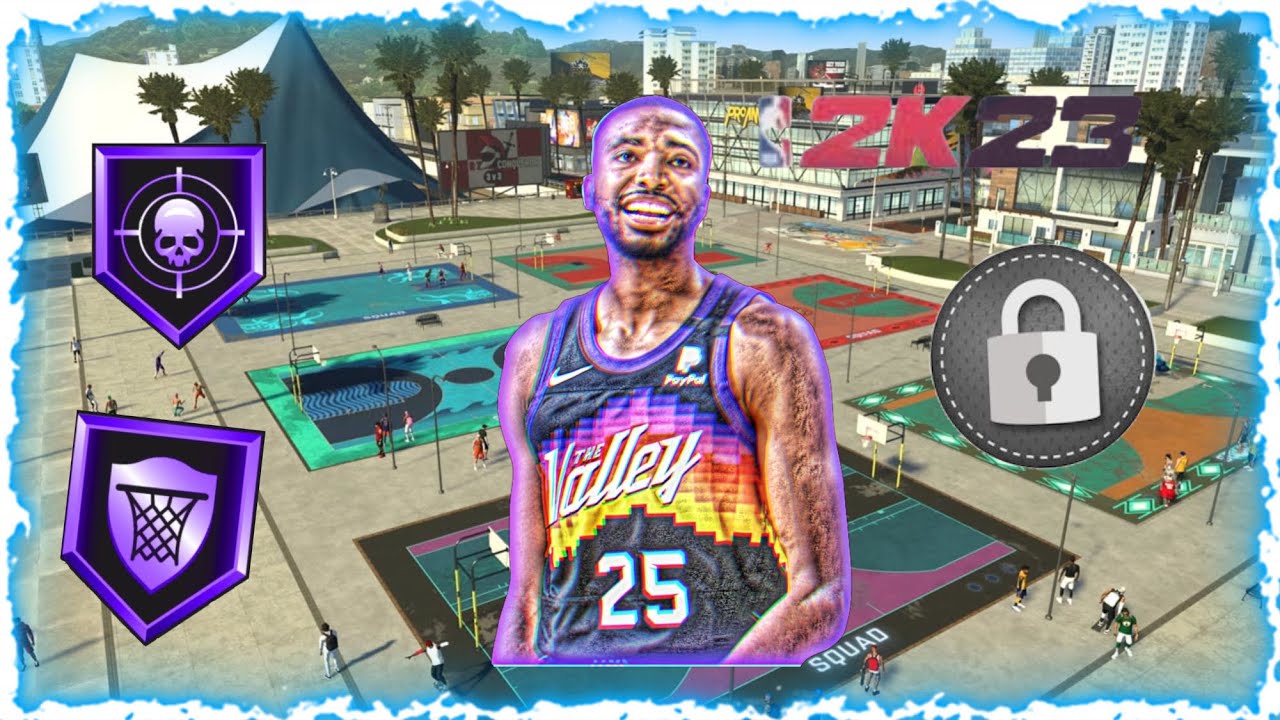This vibrant game poster for NBA 2K23 prominently features an NBA player set against a dynamic background. The color palette is a striking mixture of purple, green, yellow, and white, along with accents of brown, black, and gray, giving the scene an energetic and urban feel. The backdrop includes a mix of high-rise buildings, tents, and basketball courts, where additional players can be seen engaging in the game. The poster encapsulates the essence of NBA 2K23, merging the excitement of professional basketball with a dynamic cityscape.